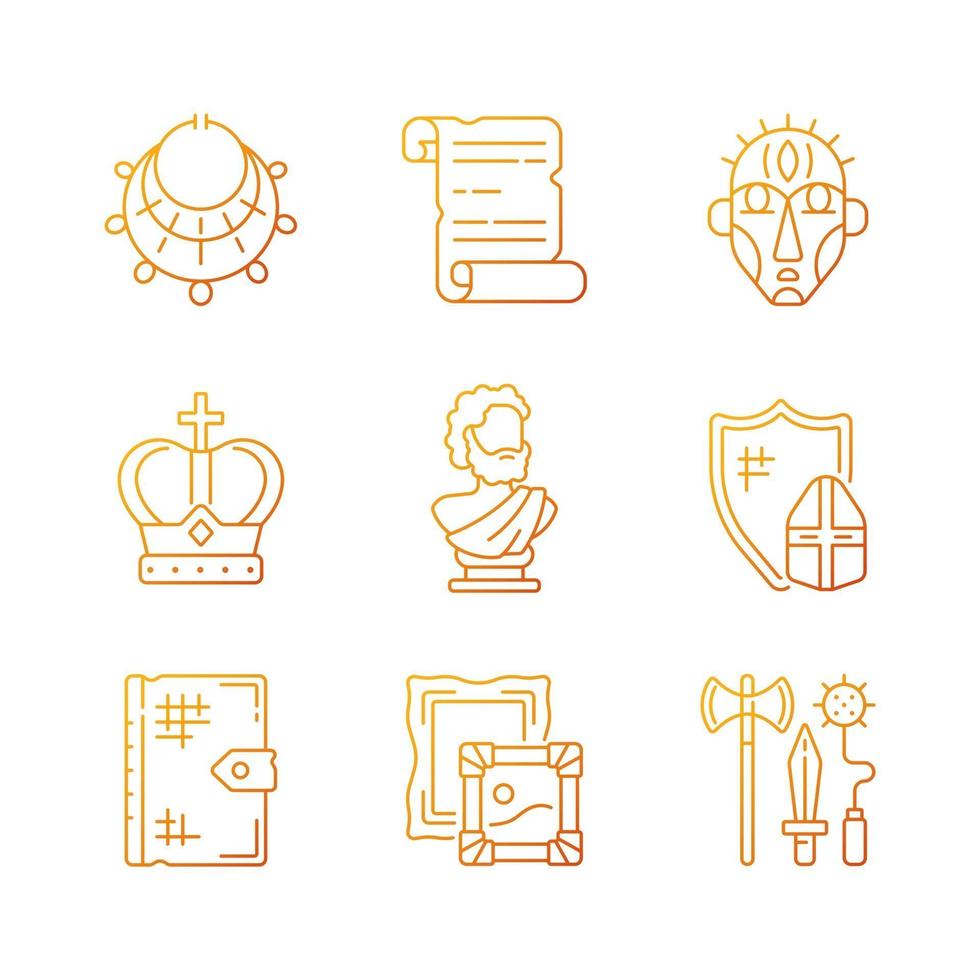The illustration showcases a series of detailed vector line arts, all set against a white background. The line art is filled with a gradient that transitions from a dark to light gold, enhancing the ornate and historical feel of the symbols. The arrangement is orderly, forming a grid of three rows with three symbols each. 

In the top row: to the left is a ceremonial necklace adorned with oval knobs, positioned in an upside-down arch; in the middle, there is an old scroll with curling ends suggestive of historical documents; and on the right, a detailed drawing of a face with hair styled like sun rays, possibly signifying a ceremonial mask.

In the middle row: to the left is a crown topped with a cross, a symbol of royal authority; at the center, there is a bust of a bearded man dressed in a toga, representing a historical figure; and to the right, a helmet paired with a shield, indicating ancient armor.

In the bottom row: on the left is a book or diary with a clasp, hinting at a secure, important document; in the middle, two picture frames of differing sizes, possibly showcasing artwork; and to the right, a collection of weapons including an axe, a sword, and a Morningstar or club with a spiked ball, symbolizing historical warfare.

This illustration could function as a set of icons in a museum, guiding visitors to different exhibits celebrating ancient and historical artifacts.